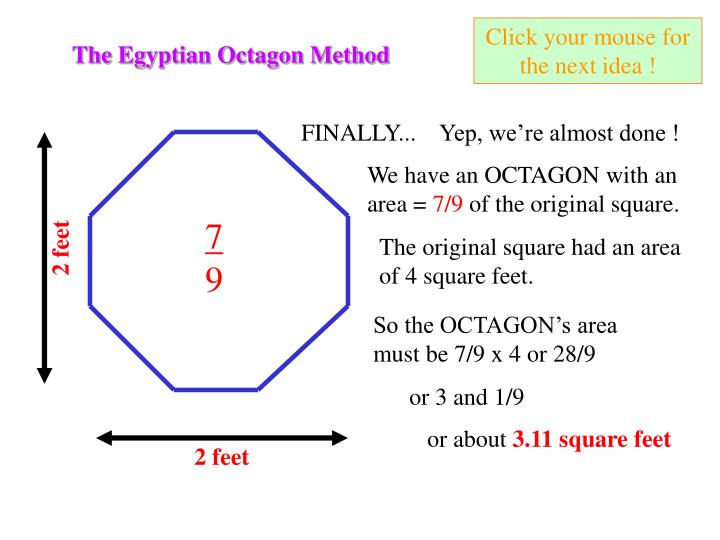The image is an infographic likely from a classroom PowerPoint presentation focused on the Egyptian octagon method. The background is white, and the content includes various geometrical shapes and textual explanations. In the top left corner, the title "The Egyptian Octagon Method" is highlighted in purple text. Adjacent to this, towards the upper right, is a green text box with yellow lettering that reads, "Click your mouse for the next idea!" Below this, there's a statement in black letters: "Finally, yup, we're almost done. We have an octagon with an area of 7/9 of the original square. The original square had an area of 4 square feet, so the octagon's area must be 7/9 times 4, or 28/9, or 3 and 1/9, or about 3.11 square feet." On the left side of the image, there is a blue octagon with the fraction 7/9 in black text at its center. Below and to the left of the octagon, two straight black arrows are shown, each annotated with "2 feet," indicating the dimensions of the octagon. Overall, this graphic seems to illustrate a geometry problem involving area calculations for a transformed shape.